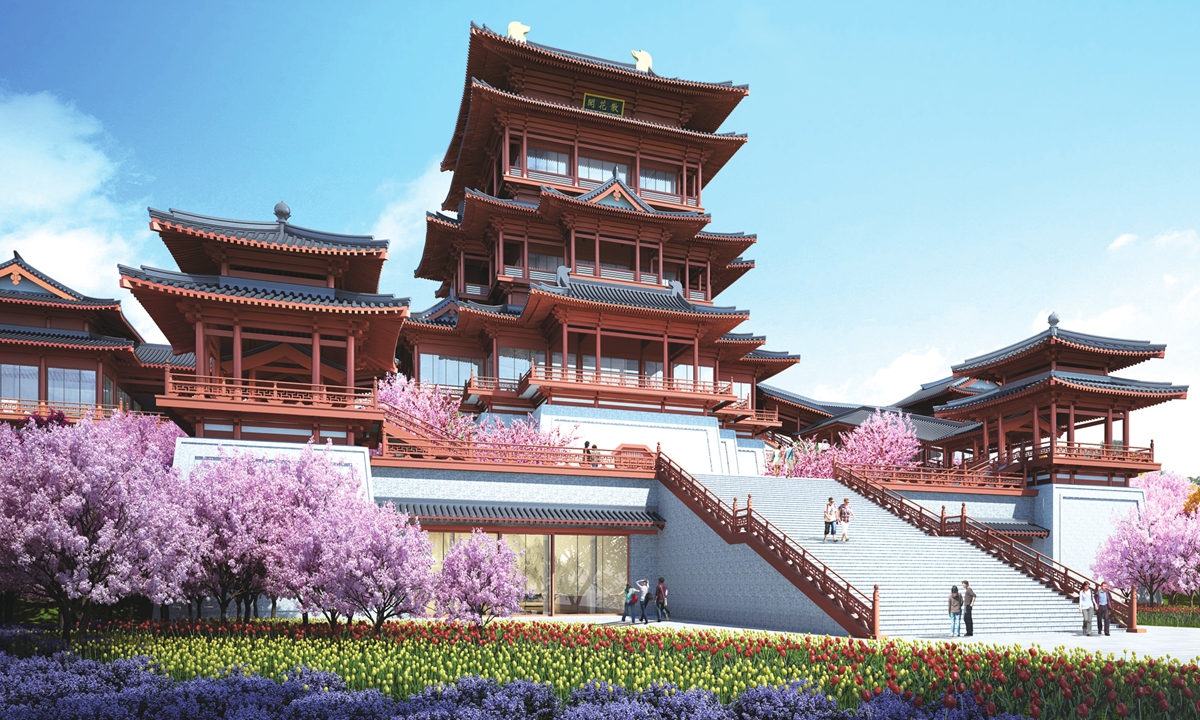This image captures a stunning, expansive Japanese pagoda, likely a temple, set against a bright blue sky on a clear, sunny day. The impressive, multi-tiered wooden structure features three prominent levels adorned with black trim, flanked by two smaller towers on either side. A sprawling gray staircase with wide, low-rise steps leads up to the second level, where several people can be seen. Surrounding the pagoda is a picturesque garden: the foreground boasts lush green grass with various smaller plants and flowers, predominantly in shades of purple, pink, and red. The first level is embraced by a plethora of trees in full bloom, their branches heavy with vibrant pink cherry blossoms. The upper levels also feature these pink-blossomed trees, adding to the overall serene and majestic ambiance of this traditional Japanese architectural marvel.